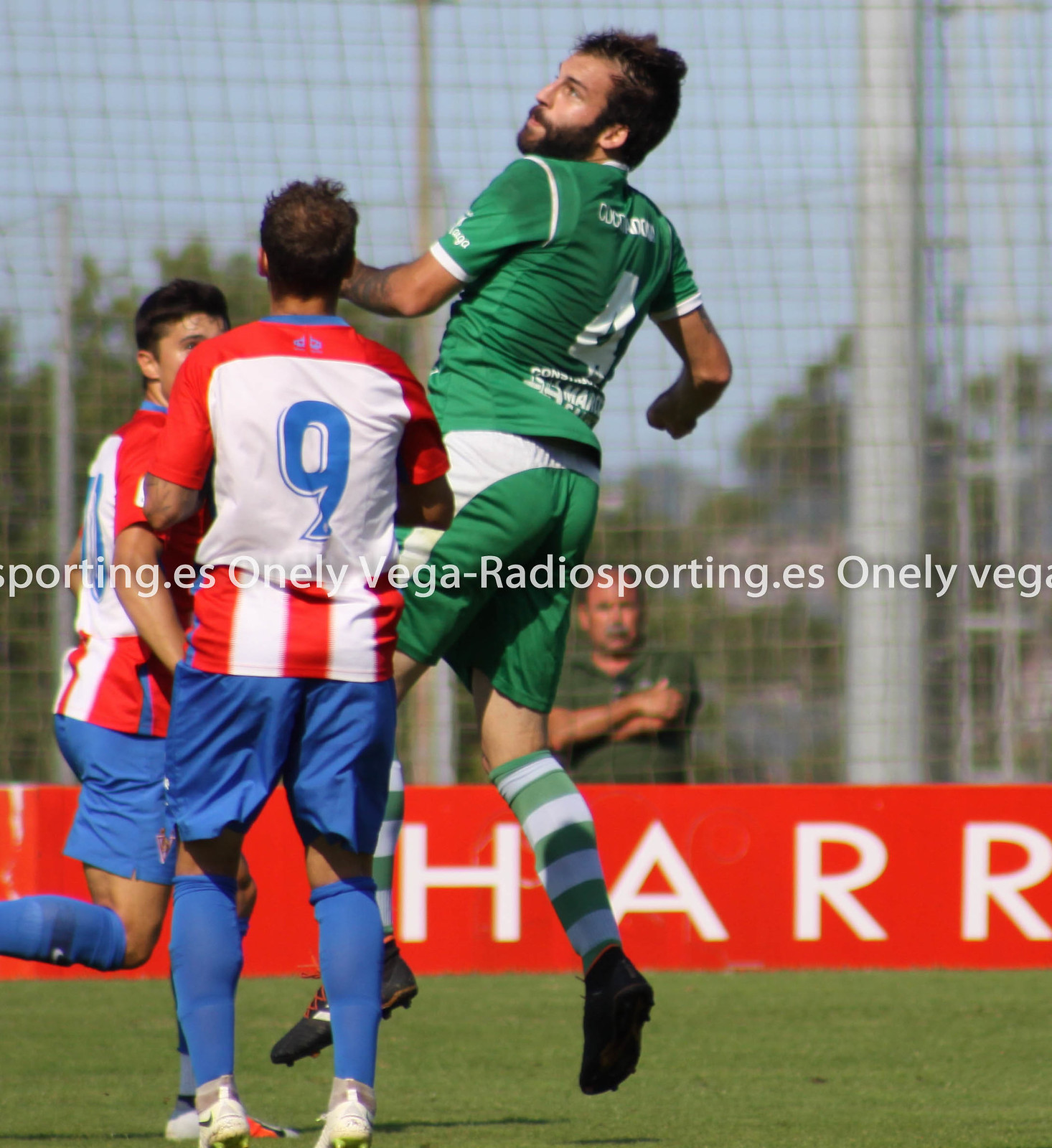In this detailed digital photograph, three soccer players are captured mid-game on a lush green soccer field, situated in front of a tall metal fence adorned with a red banner displaying the letters "H-A-R-P" in white. The central figure, dressed in a green jersey with the number 4 on his back, is caught mid-jump with both feet off the ground; his dark hair, full beard, and mustache are prominently visible along his left profile as he eyes something off-frame. This player also sports green shorts, green and white striped knee-high socks, and black cleats. 

Flanking him on the left are two teammates who don red and white jerseys paired with blue shorts and blue socks. One of these players has the number 9 printed in blue on the back of his jersey, and is turned away from the camera. In the background, a man in a dark olive green short-sleeve shirt, with arms crossed, watches the game intently from behind the fence, which is covered by a net that stretches up to the top of the photograph. Additionally, white text, seemingly part of an overlay or digital watermark, is partially visible over the top of the players, reading "OnlyVegaRadiosporting.es" in repeating segments. The colors in the image are vividly captured, showcasing a blend of green, blue, red, white, black, and gray.